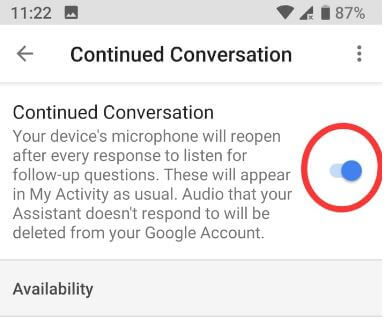In the image, a detailed notification screen is displayed outlining the settings for a "Continued Conversation" feature. At the top, in a dark gray font against a lighter gray background, the time is shown as "11:22." To the far right, the battery status is prominently indicated at "87%." Directly beneath this top bar, there is a left-pointing arrow and centered text reading "Continued Conversation."

The main body of the notification elaborates on the feature: "Your device's microphone will reopen after every response to listen for follow-up questions. These interactions will appear in My Activity as usual. Audio that your assistant doesn't respond to will be deleted from your Google account." This information is accompanied by a symbol featuring a round circle with a blue indicator at its center, presumably representing the microphone.

At the bottom of the message, the word "Availability" is displayed in dark gray text on the left side, concluding the notification. The entire message is encased within a light gray border, providing a clear and structured layout for the information presented.